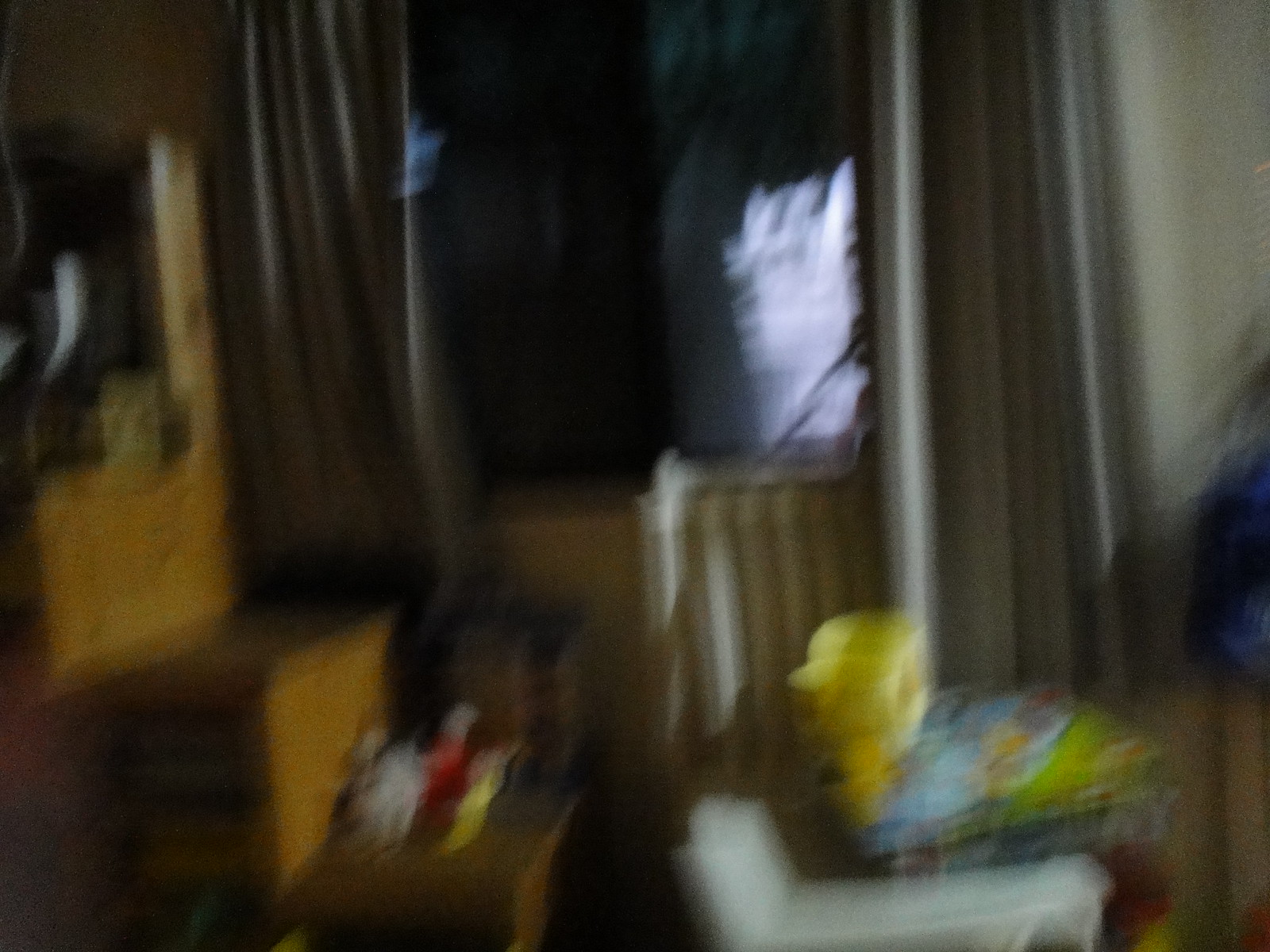This extremely blurry photograph appears to capture a living or dining room area, though precise details are difficult to discern due to the image’s poor quality. On the right side of the image, a blue, undefined shape stands out. Above and slightly to the right, a tan-colored wall is visible. Flanking either side of what seems to be a black and white window or possibly a television, there are noticeable curtain-like drapes. Below this central feature, a white object resembling a radiator is present. In front of the radiator, there is another indistinct white square form which appears to have a box atop it, characterized by yellow, blue, and green colors, potentially a board game box. To the left, there is a series of stacked brown wooden structures, possibly boxes or step-like formations, but their exact nature remains unclear amidst the blur.